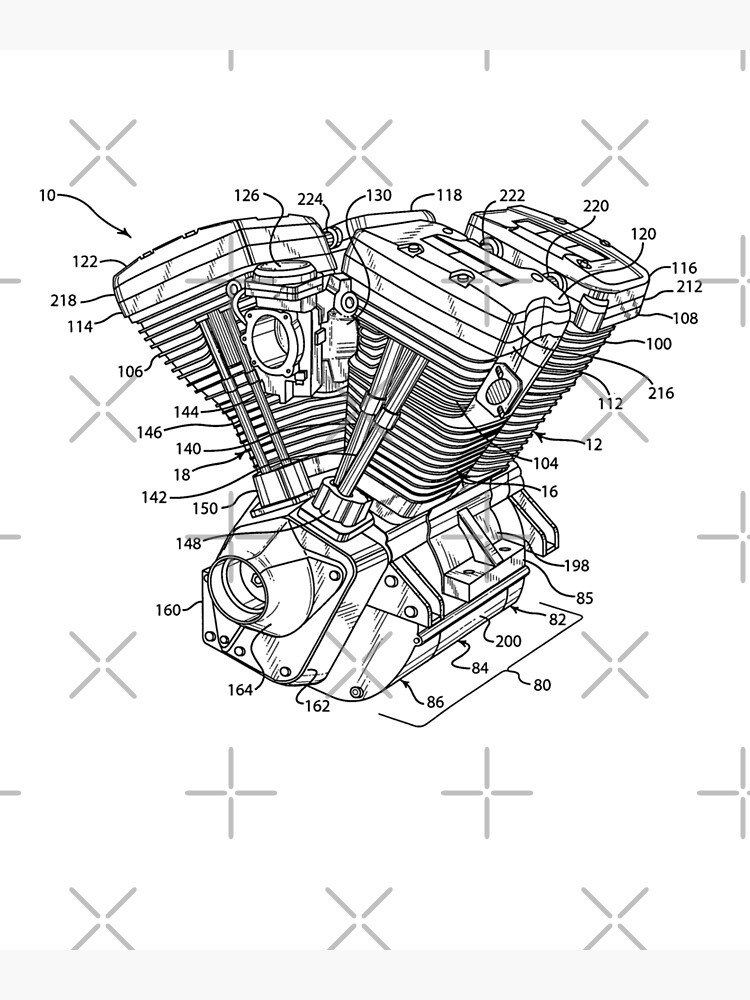This black and white illustration appears to be an informational diagram of a V-twin motorcycle engine, likely intended as a reference for mechanics. The detailed schematic features numerous lines and arrows pointing to different sections of the engine, each labeled with numbers ranging from 10 to 224, although no key or legend is provided to explain these numbers. The drawing is meticulously done, possibly by a draftsperson or engineer, and includes four prominent, vertical cylinders connected to a central crankcase, with each cylinder angled slightly away from the other. The engine sits on a base with a circular opening, suggesting where a metal bar might pass through. The image also features a distinctive watermark pattern consisting of rows of stylized X's and plus signs with their centers removed.